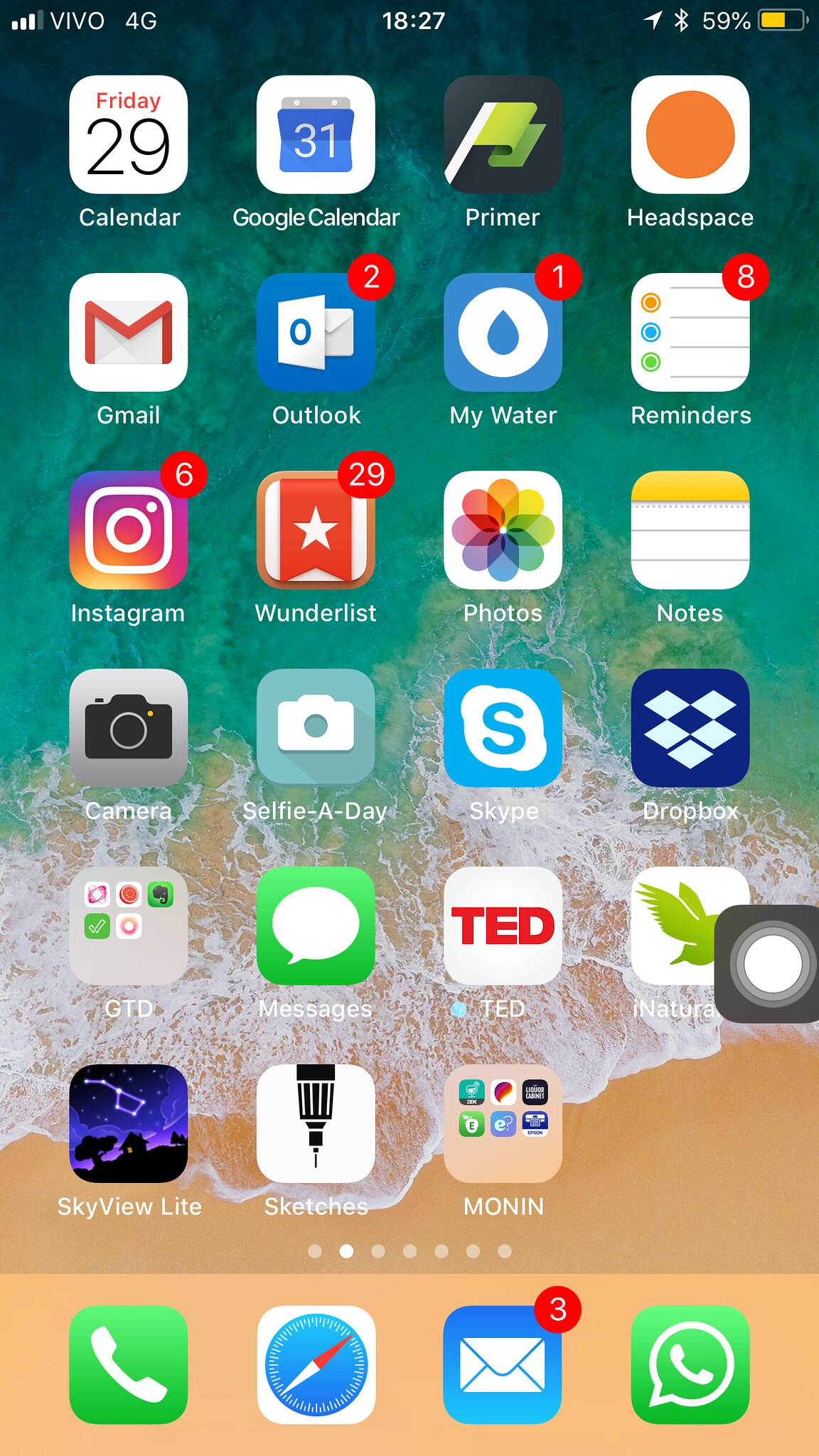A screenshot depicts a smartphone home screen densely populated with various apps, each organized in a grid pattern. The top row features organizational tools including Calendar, Google Calendar, Primer, and mindfulness app Headspace. The subsequent row showcases communication apps like Gmail and Outlook, accompanied by health tracker My Water and a Reminders app. Below, vital apps for productivity and creativity such as Notes, Photos, Wunderlist, and Instagram are arranged.

The next section includes Camera, Selfie-A-Day, and Skype, facilitating daily photo capturing and video calls. Essential storage and inspiration apps like Dropbox, a Nature app, TED app, occupy the following row. There's also a Messages app for texting, a GTD (Getting Things Done) app featuring a folder with five sub-apps, Skyview Light for stargazing, and Sketches for drawing enthusiasts.

At the bottom of the screen, vital utility icons are located: the traditional green Telephone app, Compass for navigation, and the well-known Messages app for texting, alongside an additional phone-related app featuring a green icon with a telephone symbol inside a circle with a triangle, possibly indicating another messaging service. Lastly, an email app represented by an envelope icon completes the organized display of versatile applications.